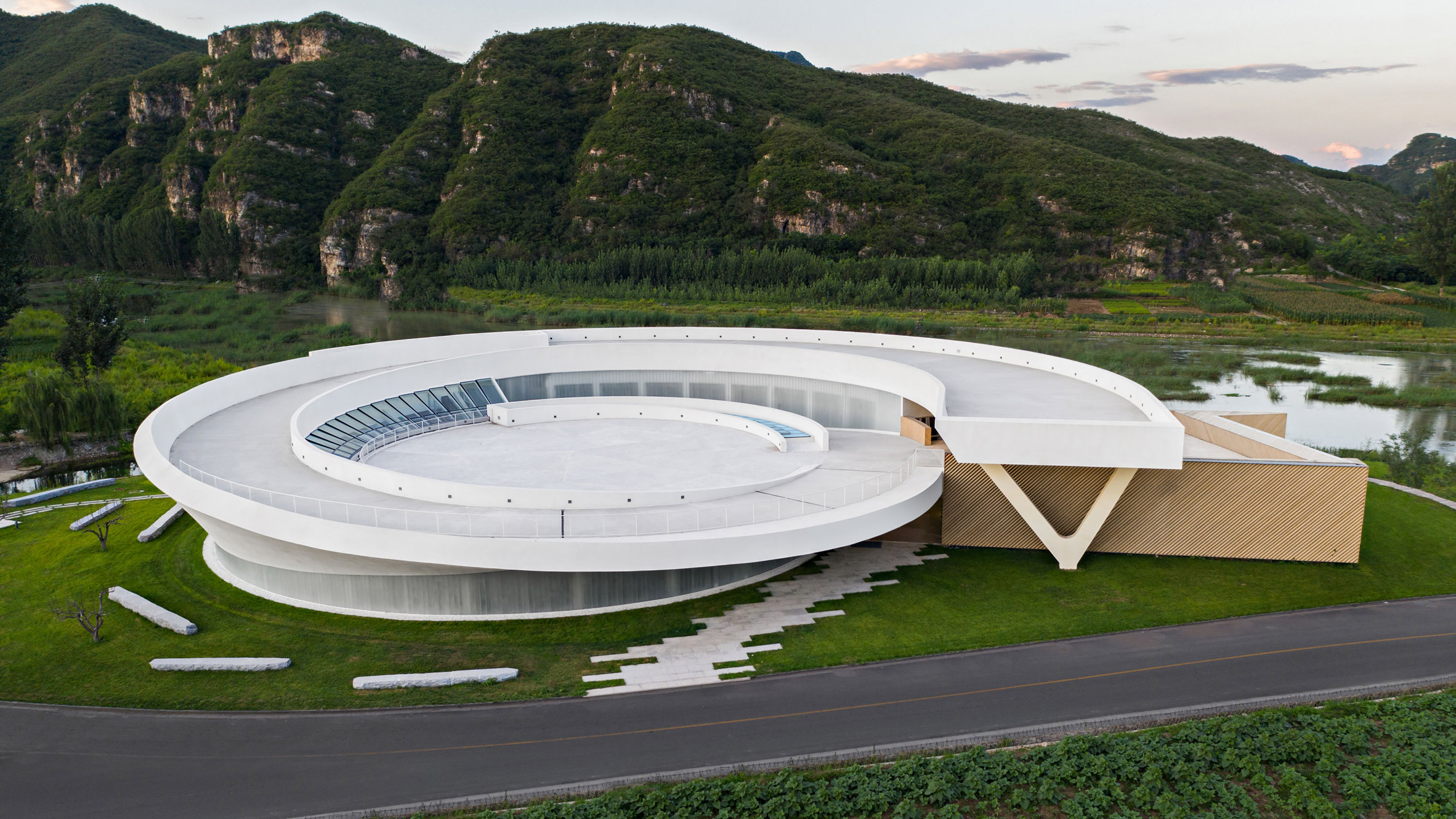The image captures a stunning piece of modern architecture positioned in a vast grassland valley, with rugged, tree-covered mountains towering in the background. The time of day appears to be evening, as the sun is nearing the horizon, casting a soft light across the landscape. An aerial perspective reveals the building's intricate white structure featuring a unique spiral ramp that encircles once before merging into another wall. The building is supported by a V-shaped brace at its base and also incorporates a light brown, tan-colored addition extending from the right side. A shallow body of water lies in front of the mountains but behind the building, enhancing the serene setting. The area includes scattered slabs of white concrete, forming a path leading toward the architecture while some are randomly placed on the green grass. A black paved road runs in front of the building, completing the scene of this remarkable and very modern architectural spectacle.